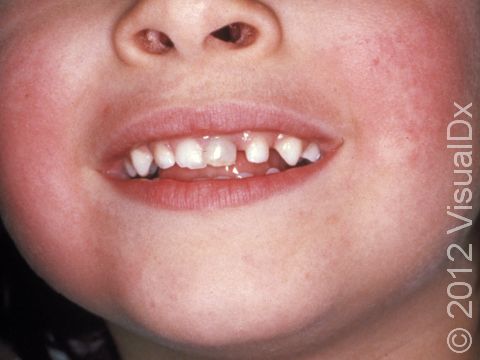The image is a horizontal, rectangular photo taken in landscape orientation, showcasing a close-up of a child's face from the nose down, focusing on their open mouth in a light smile. The child has visible nostrils, cheeks, lips, chin, and the top of their neck. Their teeth are prominently featured, revealing gaps and uneven spacing, suggesting the need for orthodontic work such as braces. The skin appears youthful, wide, and pink with flushed cheeks, giving an overall impression of a child's face. A vertical watermark on the right side reads "© 2012 visual DX."